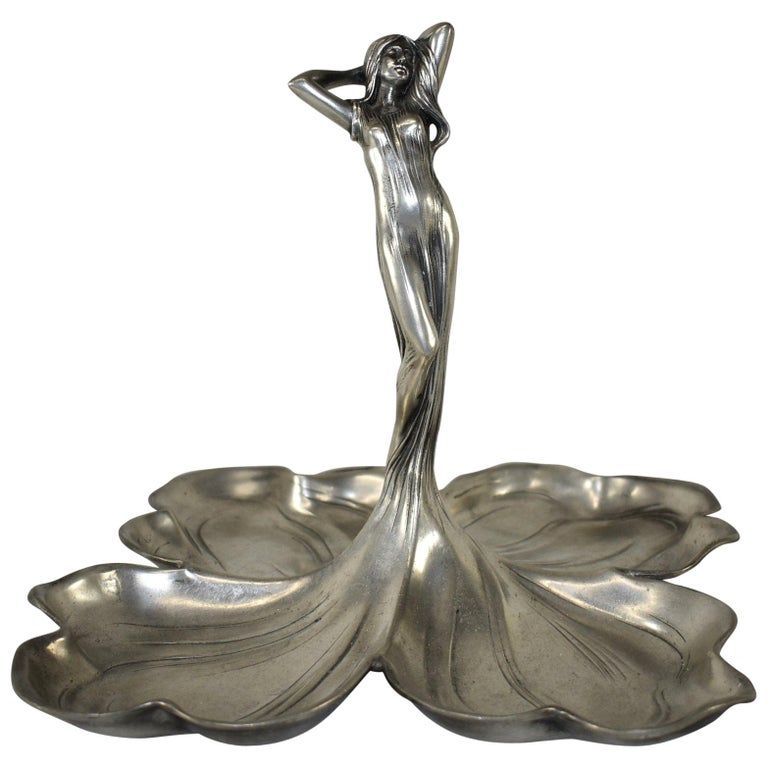The photograph features a meticulously staged, monochrome image of a silver metallic statue of a very slim woman. Set against a plain white screen background, the statue's finely detailed craftsmanship suggests it might be composed of pewter or silver. The woman is depicted with long, flowing hair cascading down to her shoulders, and she elegantly poses with her arms raised and hands positioned behind her head, tilting her face gently against her left arm. 

Her form-fitting, intricate dress flows down from her shoulders and seamlessly spills out towards the base, creating four distinct petal shapes that resemble shells or a clover pattern when viewed from above. These petal-like extensions at the base are akin to small containers or trays, adding a functional yet artistic element to the piece. The statue as a whole exudes a sense of grace and fluidity, reminiscent of a stylized art trophy or decorative artwork.